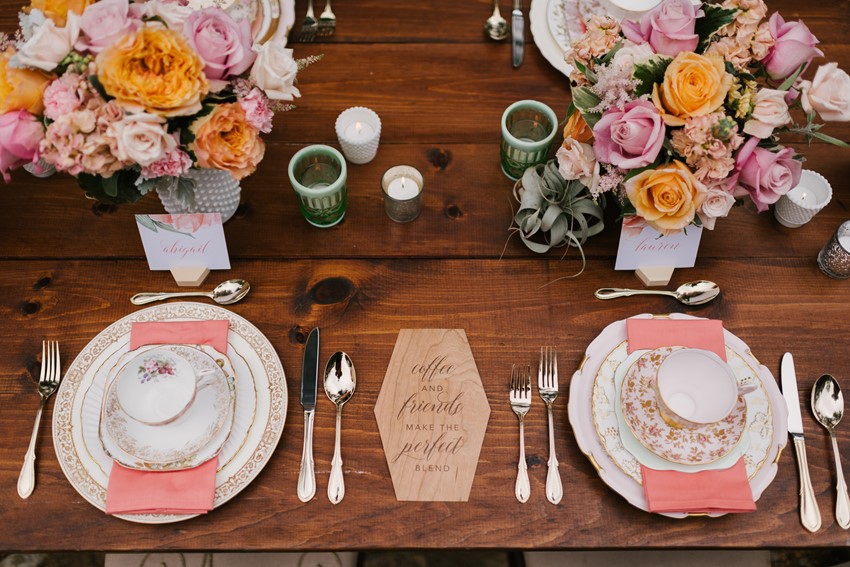This aerial view captures a beautifully set dinner table on a refurbished wooden surface, adorned with delicate and colorful floral arrangements and intricate dinnerware. Two elegant bouquets feature a variety of flowers, including pink, orange, and yellow blooms, and are placed in vases at either end of the table that bear the names Abigail and Lauren. Central to the table setting are small green votive candles and assorted seasoning shakers, creating a warm and inviting ambiance.

Each place setting includes a larger plate, a smaller plate, and an intricately designed flowered coffee cup perched on a pink napkin. Above each plate setting lies a visually appealing arrangement of silverware: two forks to the left and a knife and spoon to the right. There is a decorative placemat that reads, "Coffee and friends make the perfect blend," underscoring the cozy and welcoming atmosphere of the scene. The entire setup, viewed from above, highlights the meticulous attention to detail and the intention for an intimate and sophisticated dining experience.